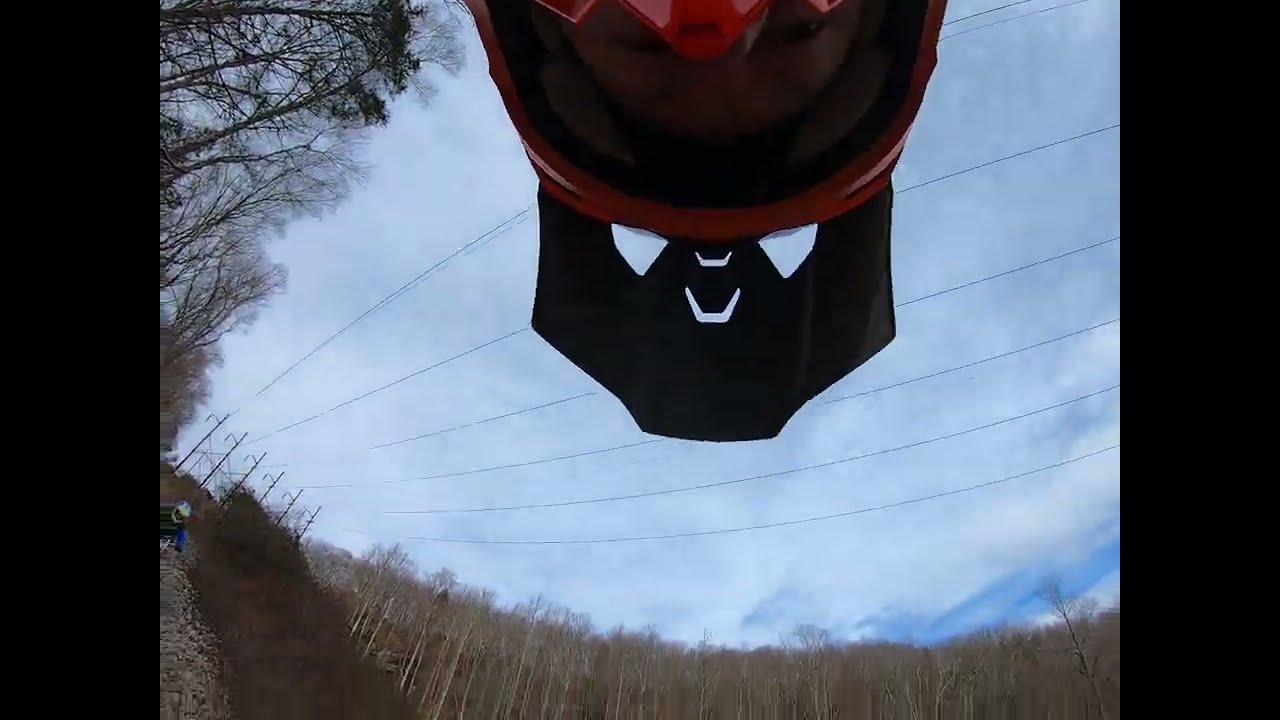This rectangular photograph is approximately 3 inches tall and 6 inches wide, with black vertical bars framing the left and right edges, each about an inch wide. The outdoor daytime scene captured in the center shows a cloudy sky with patches of blue. Six power lines extend diagonally from the lower left to the upper right, intersecting with a row of telephone poles. Emerging from the top center of the image and appearing upside down is a face of a Caucasian person wearing a full-faced, red helmet with a black visor that has holes, resembling a humorous smiley face. Below, the barren tree line stretches across the width of the image with trees devoid of leaves, and in the lower left corner, a cyclist in blue, wearing a white helmet, is seen riding towards the camera.